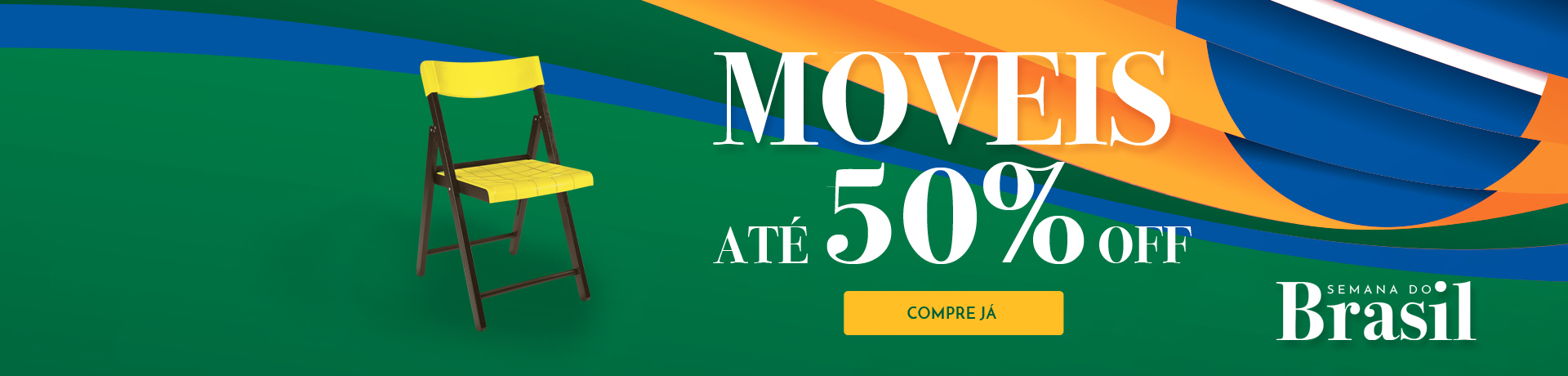The digital advertisement banner features a vivid depiction with primary colors of green, blue, yellow, and orange, prominently emulating the Brazilian flag. Central to the left of the image is a yellow foldable chair with brown legs, casting a slight shadow, which appears computer-generated. The chair is positioned not entirely to the left but more towards the middle left of the composition.

In the background, there is a stylized rendition of the Brazilian flag characterized by a textured blue circle, with a layered gold, white, and green design swirling from left to right. The main promotional text is centered and reads “Móveis até 50% off,” indicating a 50% off sale on furniture. Additionally, a yellow button with green font underneath the main text says "Compre já," suggesting an actionable click.

At the bottom right, there is another text in white letters on a green background stating “Semana do Brasil,” highlighting the promotional week. The composition suggests a festive and vibrant sale advertisement, invoking Brazilian patriotic elements amidst a colorful and engaging layout.